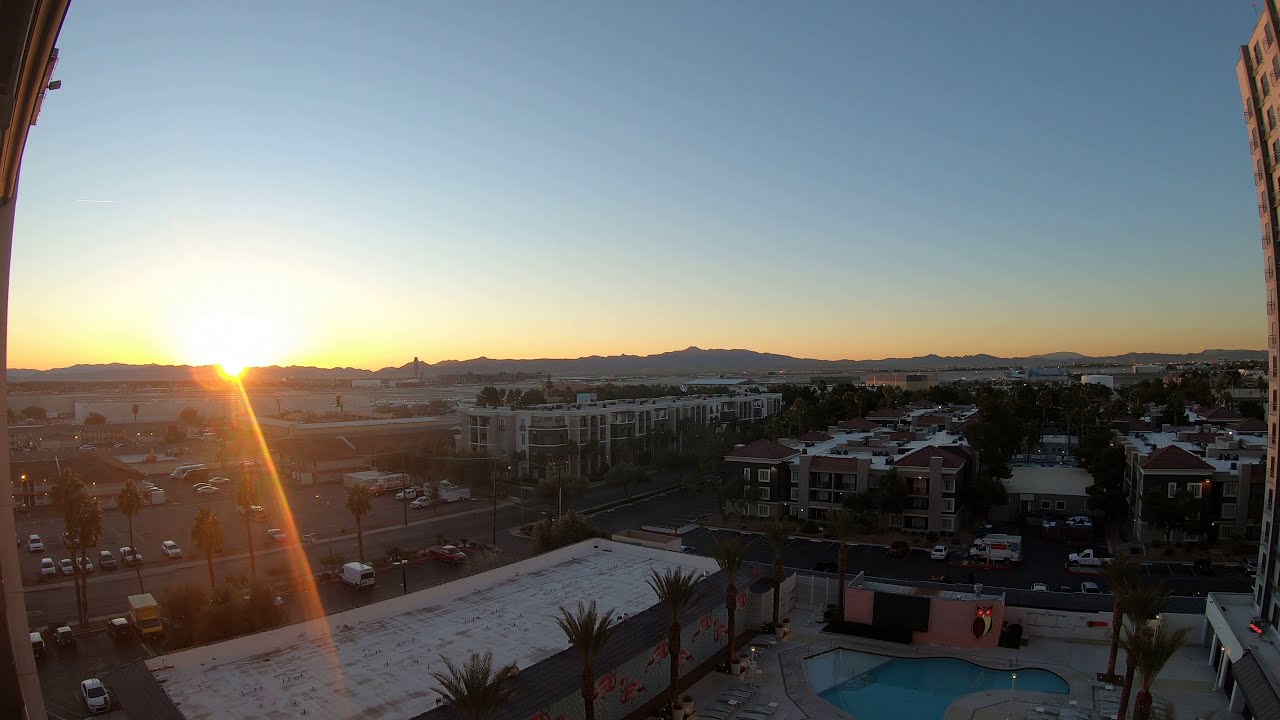The image captures a cityscape at dusk, with the sky transitioning from blue to hues of orange and yellow as the sun sets behind a distant mountain range. In the far background, the mountains stretch across the horizon, with the sunset's rays casting a warm glow. To the left, a vast parking lot filled with numerous parked cars lies adjacent to the mountains. On the right side of the image, several residential and commercial buildings, including a tall apartment building, rise prominently. Near the bottom right of the image, there's an irregularly shaped swimming pool, bordered by palm trees and fitted with lights, though it appears empty of people. A nearby building features a distinctive image of an owl with bright red eyes. The image as a whole encapsulates a tranquil evening in a bustling city, with its blend of natural and urban elements illuminated by the setting sun.